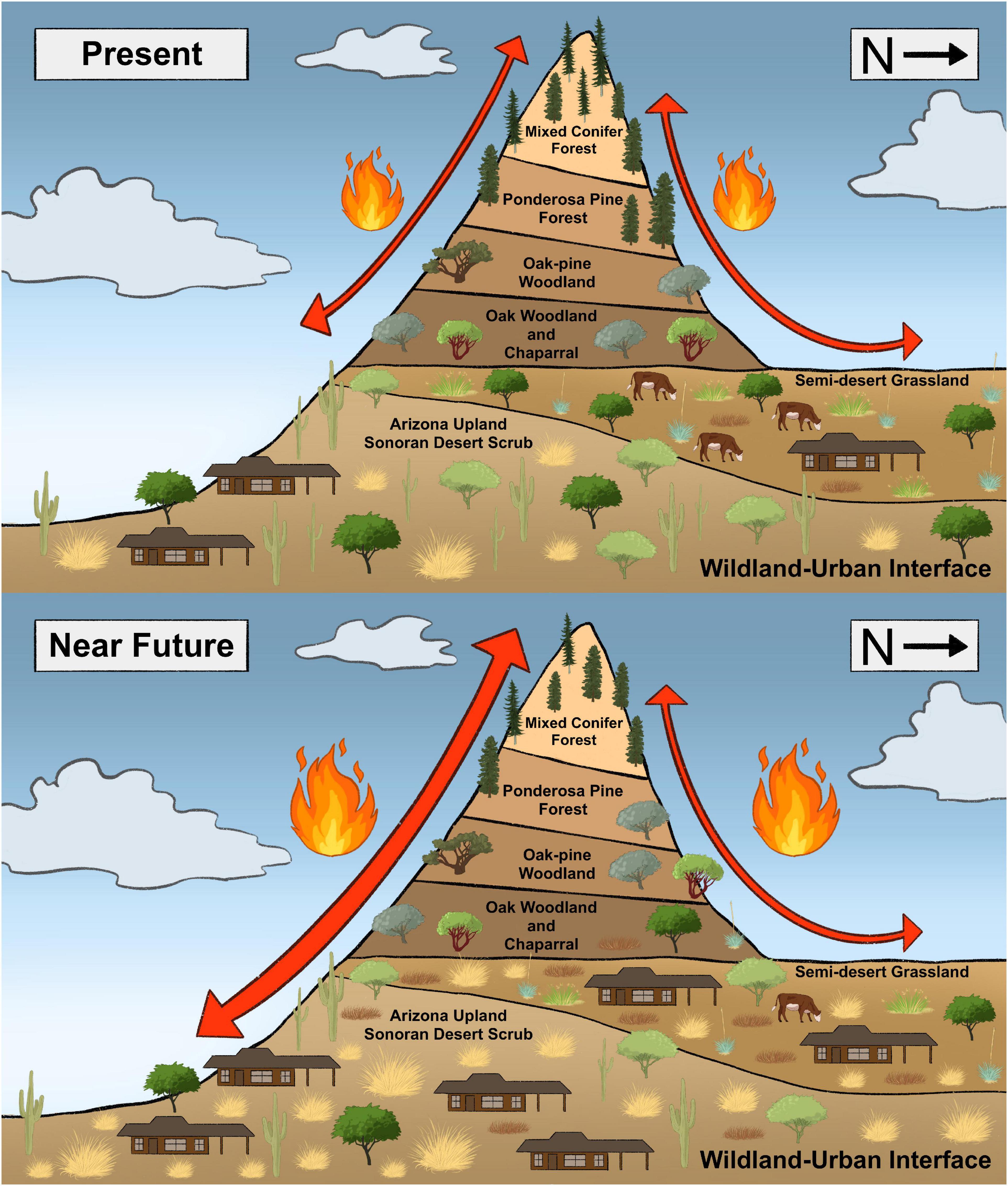The image depicts a detailed diagram of a mountainous wildland-urban interface, illustrating the impact of wildfires over time. The top half of the illustration, labeled "Present" in a white box with black text, showcases a mountain with segments of vegetation, including mixed conifer forest, ponderosa pine forest, oak pine woodland, oak woodland and chaparral, semi-desert grassland, and Arizona upland Sonora desert scrub from top to bottom. The sky is blue with three white clouds, and to the top right, there is an 'N' with an arrow pointing to the right.

On the mountain, several elements are depicted: three buildings scattered around, a stable with three cows, and various trees and cacti. Each side of the mountain is marked with red arrows pointing up and down, accompanied by flame icons indicating the presence of fire dynamics.

The illustration's bottom half, tagged "Near Future" in a blue box with black text, depicts the same landscape but with noticeable changes. Some trees are missing, and the wildlife is reduced to one cow, while the flame icons next to the red arrows are significantly larger, indicating increased fire activity.

Both diagrams are labeled 'wildland urban interface' in the bottom right corner, elucidating the potential progression of wildfires and their impact on this region.